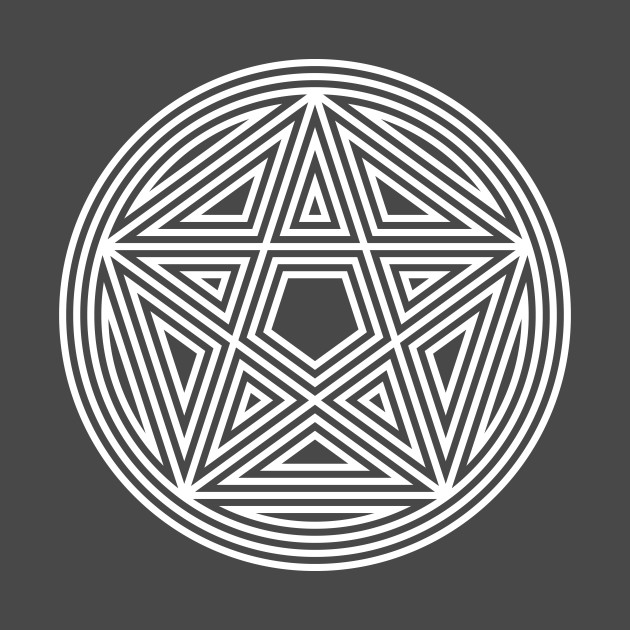The image depicts an ornate and intricate pentacle or pentagram design against a medium light gray background. At the center, a small solid black pentagon anchors the composition. Surrounding this are multiple layered geometric shapes, filling the negative space with triangles and additional pentagons, enhancing the visual complexity. The main feature is an upright five-pointed star inside a larger pentagon, itself situated within three concentric circles. The entire design employs white lines to create this web of shapes, resulting in a psychedelic and embossed effect, blending the star and circular motifs seamlessly together.